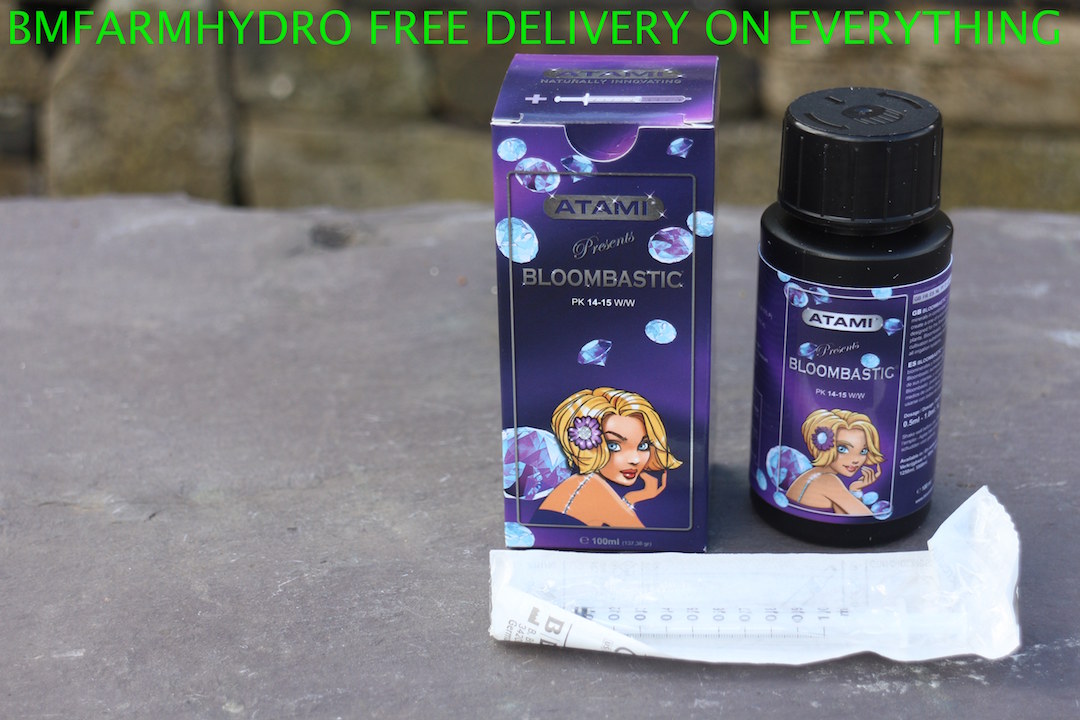In this photograph, a small black bottle is positioned on a gray, stone-like surface. Attached to the bottle is a purple label featuring the text "Atami" and "Bloom Bastic," along with an illustration of a woman. To the left of the bottle stands its cardboard container, which is also purple and displays the same text and artwork. In front of the bottle and its container lies a white paper receipt. At the top of the image, green capital letters spell out "BM Farm Hydro, free delivery on everything." This detailed composition highlights the product and its packaging while promoting the brand's delivery service.